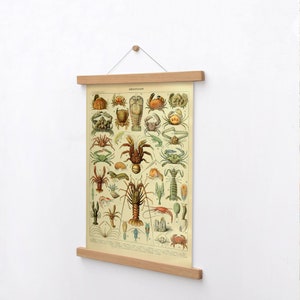Hanging on a stark white wall is a decorative scroll-like poster, suspended from a brown pushpin by a string. The poster itself has wooden rectangular bars at the top and bottom for weight, allowing it to hang smoothly. The background of the poster is a very light green color, providing a subtle contrast against the wall. Displayed prominently on this poster are various illustrations of marine life, predominantly showcasing different types of crustaceans such as crabs, lobsters, and shrimps. These creatures are rendered in a diverse palette, including orange, green, pink, and brown. Arranged in a manner reminiscent of a scientific diagram, the poster features around 25 different species, displayed side-by-side in a textbook-like format. Although there are words at the bottom of the poster, they are too small to read from a distance.